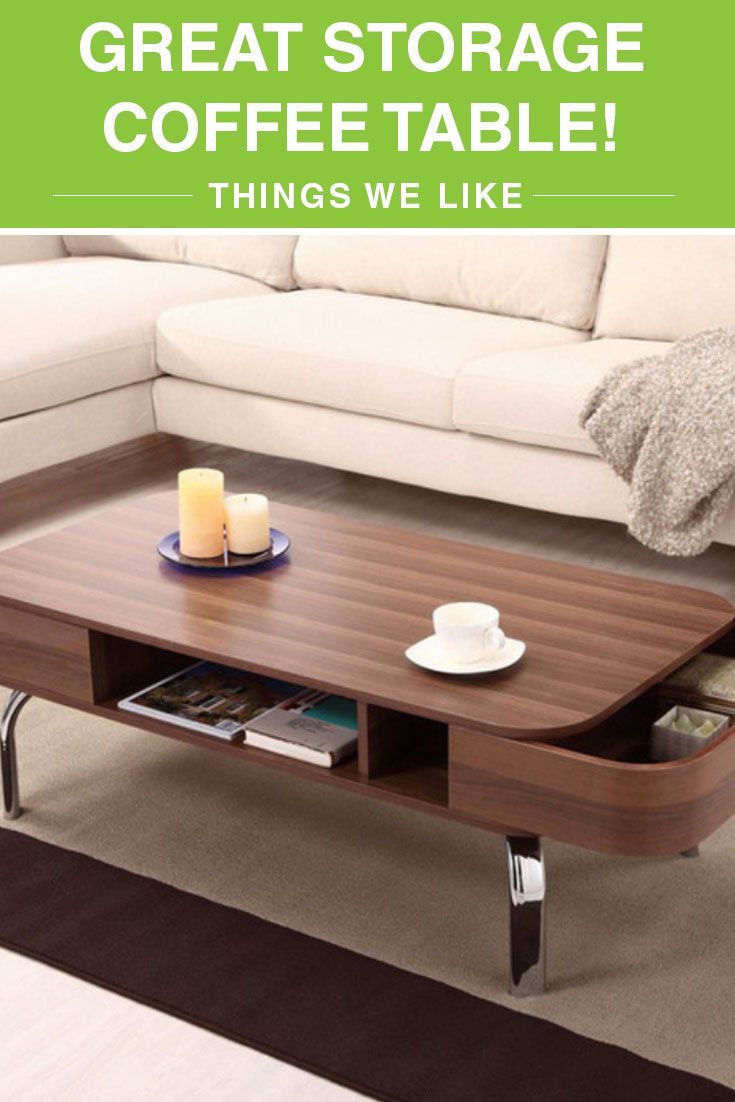This advertisement image showcases a stylish and modern interior design. Central to the composition is a diagonally-placed white sectional couch with a gray sweater draped over one end. In front of the couch, positioned on a beige rug, is an elegant brown wooden coffee table with polished metal legs. The coffee table, which features convenient storage shelves beneath and side drawers for additional storage, is adorned with a variety of items: a small square white saucer with a coffee cup, and a blue plate holding two beige candles of differing heights. At the top edge of the image, a green rectangle contains the following text in all-caps white lettering: "GREAT STORAGE, COFFEE TABLE, THINGS WE LIKE."